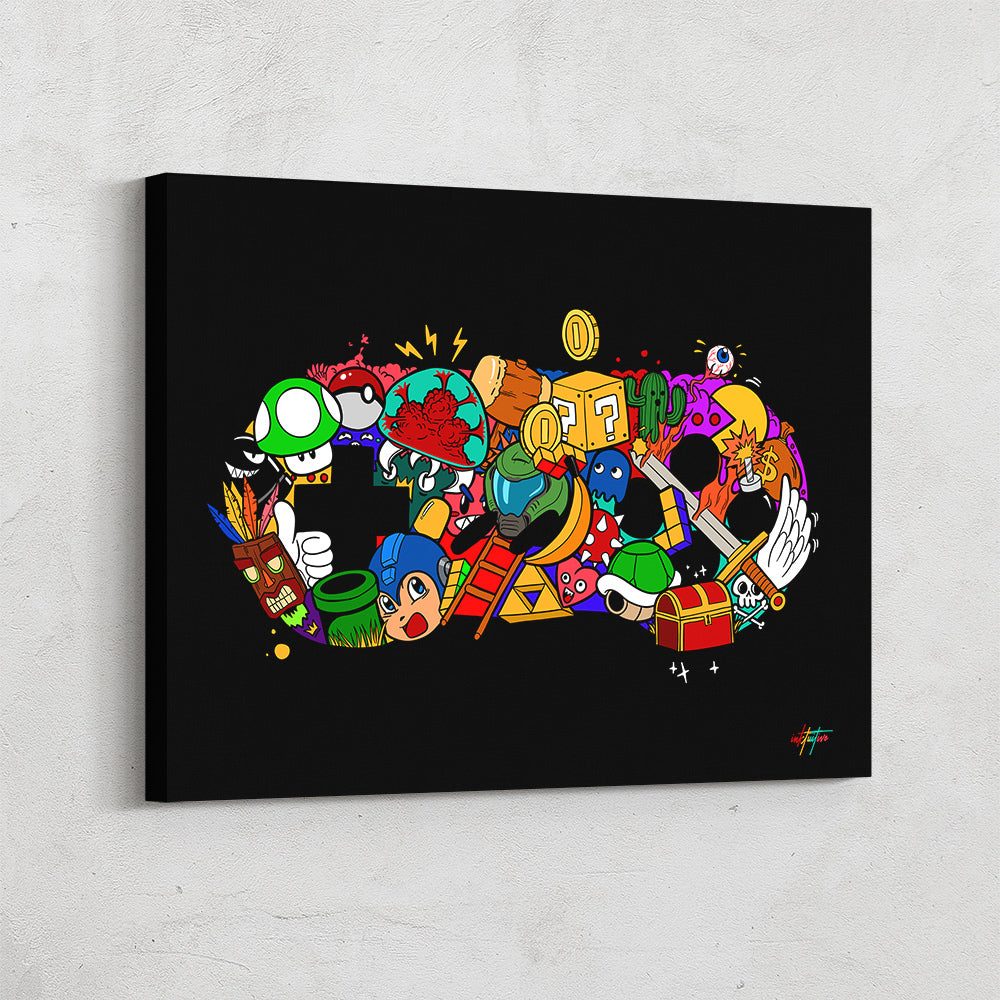This wall art illustration, framed on a black canvas board, bursts with vibrant colors such as orange, blue, yellow, red, white, green, pink, and purple. The artwork meticulously combines elements from various video games spanning decades, arranged in an intricate design resembling a gaming controller, potentially a PlayStation one. Within the oval-shaped collage, you can identify iconic gaming symbols: a treasure chest, Pac-Man ghosts, question mark dice, a money bag with a dollar sign, golden coins, Super Mario Brothers mushrooms, a heart with eyes, a ladder, Sonic's head, a Rubik's Cube, a tiki mask, a brain within a bubble, a barrel, a cactus, an eyeball, a turtle shell, a wing, a sword, and a thumbs-up hand. Additional notable elements include a Pokemon ball and Donkey Kong components. This piece exudes a retro 1980s vibe. At the bottom-right corner, a colorful signature—composed of red, yellow, and aqua blue colors—decorates the artwork, although the exact text of the signature remains indiscernible. The black canvas itself rests against a light gray wall, presenting a visually dynamic homage to video game history.